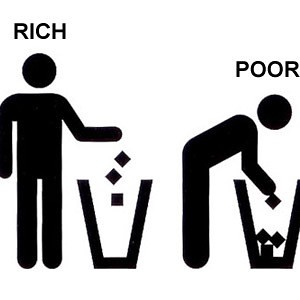The image is a computer-generated graphic featuring two black stick figures against a white background, each labeled "rich" and "poor," respectively. Both figures have detached circular heads and are set next to a garbage can. The figure on the left, labeled "rich," stands upright, throwing three pieces of paper into the trash. On the right, the figure labeled "poor" is bent over, picking one of the four items from the garbage can, which is partially cut off at the edge of the image. This visually striking image serves as a social commentary on wealth disparity, illustrating how the rich discard items that the poor must scavenge for survival.